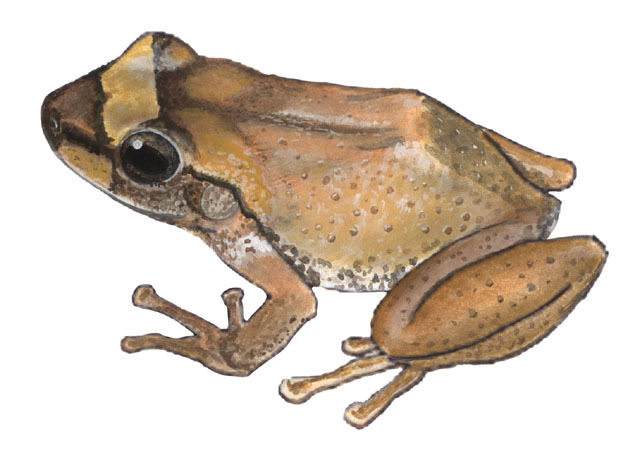The image depicts a highly detailed, realistic illustration of a small frog rendered in a mixture of brown, olive, taupe, and beige tones, with hints of yellow and green. The illustration, likely a colored pencil drawing or painting, showcases the artist's meticulous attention to detail in capturing the frog’s expressive face and intricate coloring. The frog is shown from a side profile, perched on all fours with its three-toed feet visible, almost giving the impression of readiness to leap. Its wary, expressive eye suggests a sense of unease under scrutiny. Placed against a plain white background, the image has been digitally isolated, possibly using Photoshop, to remove any distractions and focus purely on the charming and lifelike depiction of the frog.